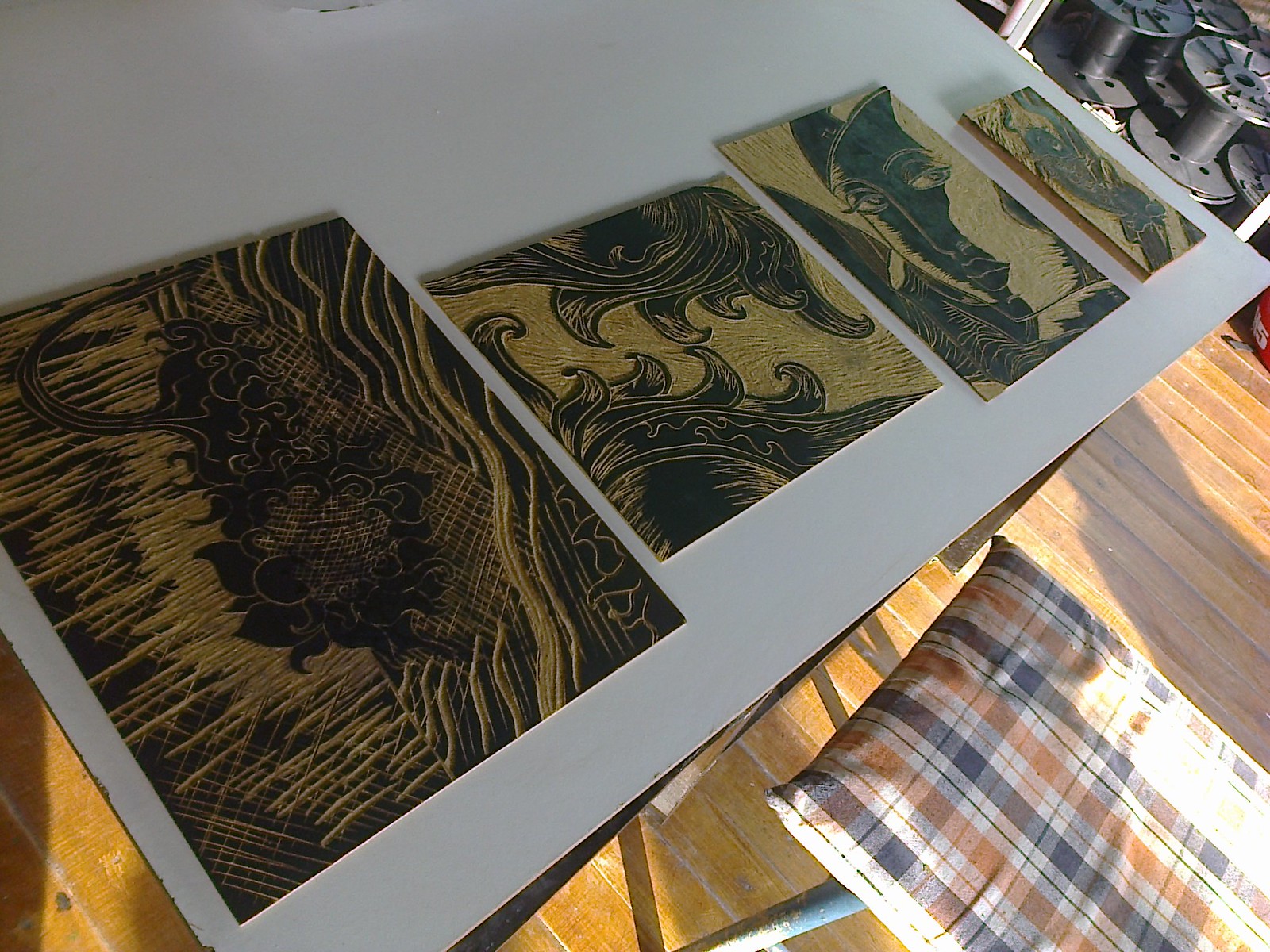This detailed full-color photograph, taken in an indoor setting, captures an art display on a hardwood floor bathed in natural sunlight. Splitting the image diagonally, the top half reveals a white table positioned slightly from the bottom left to the top right, showcasing four horizontal pieces of artwork with gold and black tones. In the far top-right background, four empty black wire spools are visible. In the bottom right, to the side of the table, stands a small stool featuring a plaid cushion with blue, orange, and white colors. Surrounding these objects, the floor showcases shades of white and brown, adding a rustic contrast to the scene's overall calm and creative ambiance. A light blue hue from the stool complements the earthy palette, enhancing the intimate display of handcrafted artwork.